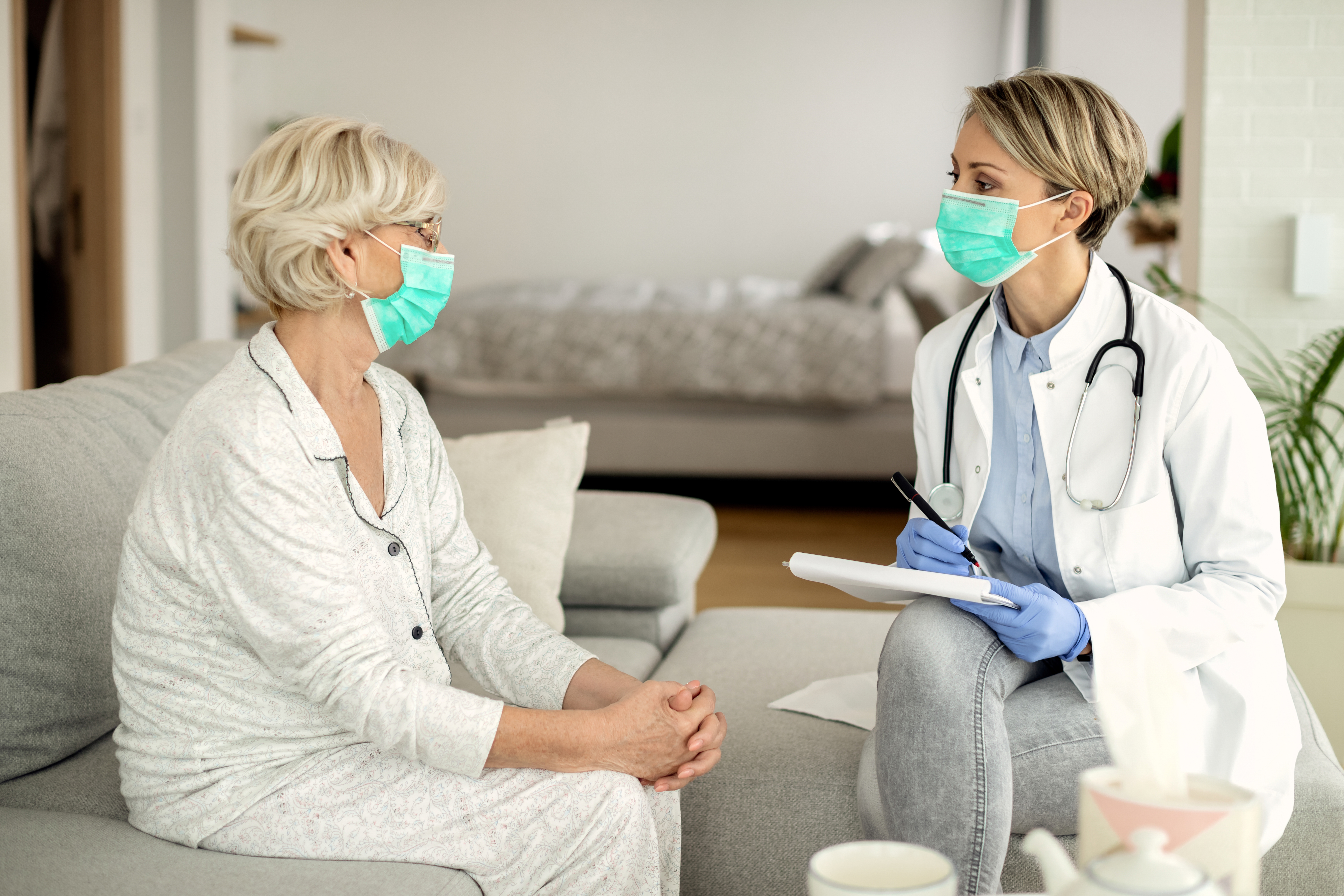In a brightly decorated, well-kept room with white walls and polished wood floors, two women are engaged in conversation, suggesting an in-home medical consultation. The room, which features a bed against the wall, plants, a closet door, and an inviting cup of tea in the foreground, evokes a sense of warmth and care, akin to an assisted living environment. One woman, an elderly patient with grayish blonde hair, glasses, and dressed in pajama-like attire, sits on a small sofa, donning a face mask. Next to her, positioned on an ottoman upholstered in matching fabric, sits a healthcare professional in her late 30s to early 40s. She is identifiable by her white doctor's coat, stethoscope around her neck, blue button-up blouse, gray skinny jeans, and blue rubber gloves. Her short blonde hair peeks out from behind a seafoam green face mask. Holding a notepad and a pen, the doctor appears attentive as she converses with the patient, capturing the essence of a compassionate and personalized home visit.